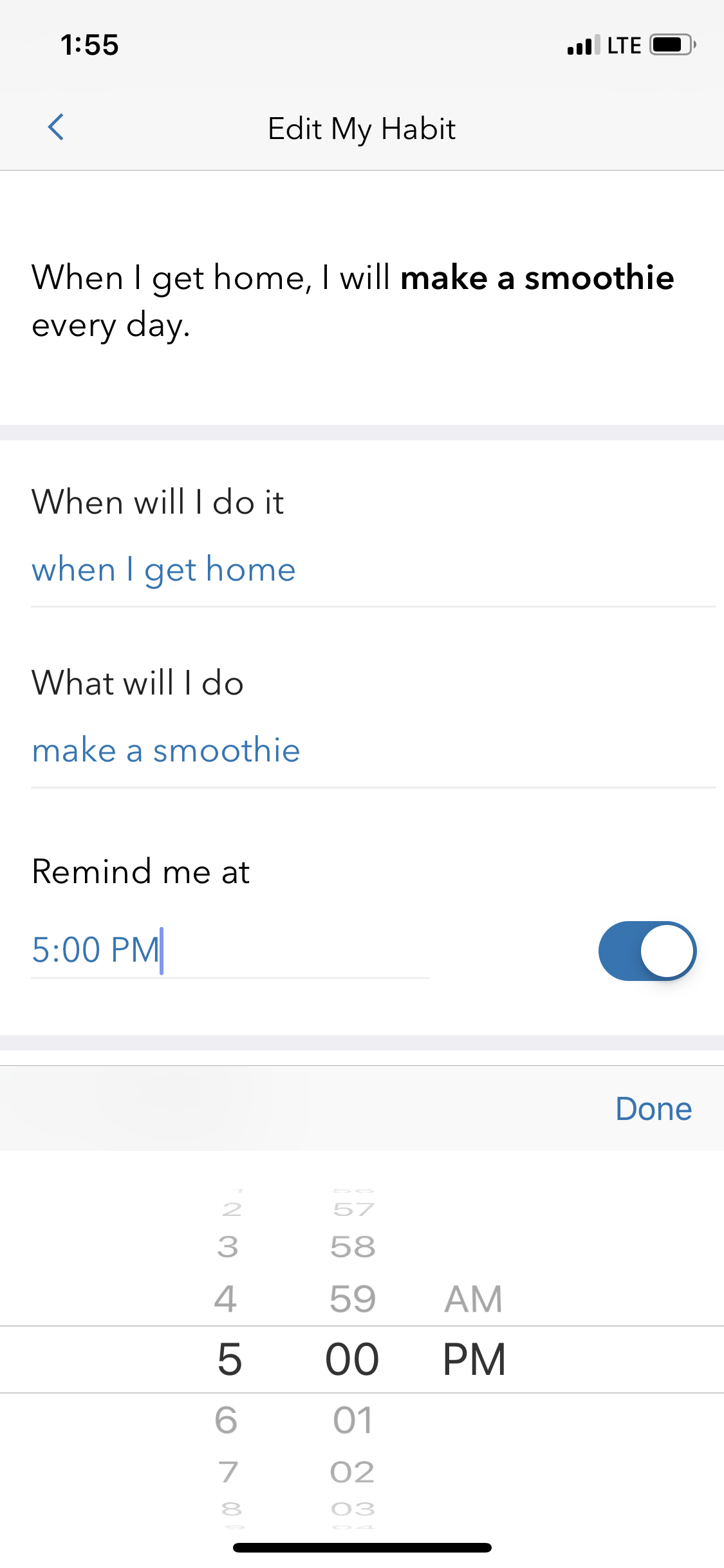On an iPhone screen displaying a website, the battery life indicator shows approximately 75% charge, and the device time is 1:55 PM. The phone is connected to LTE. The webpage titled "Edit My Habit" is framed within a grey box at the top of the screen. Below this, in a white section, the text reads, "When I get home, I will make a smoothie every day."

A light grey bar separates this from the next section, which asks in blue text, "When will I do it?" The corresponding answer, "When I get home," is also in blue. Further down, another prompt in blue asks, "What will I do?" with the reply, "Make a smoothie," also in blue. Beneath this, the text "Remind me at" is shown with the time set to 5:00 PM, highlighted in blue. 

There is a blue slider next to the reminder time, indicating the reminder is active. The time setting section functions similarly to the standard time-picker on the iPhone, allowing the user to scroll to select the hour and minute, and toggle between AM and PM. The black bar at the bottom of the cell phone screen signifies the end of the webpage.